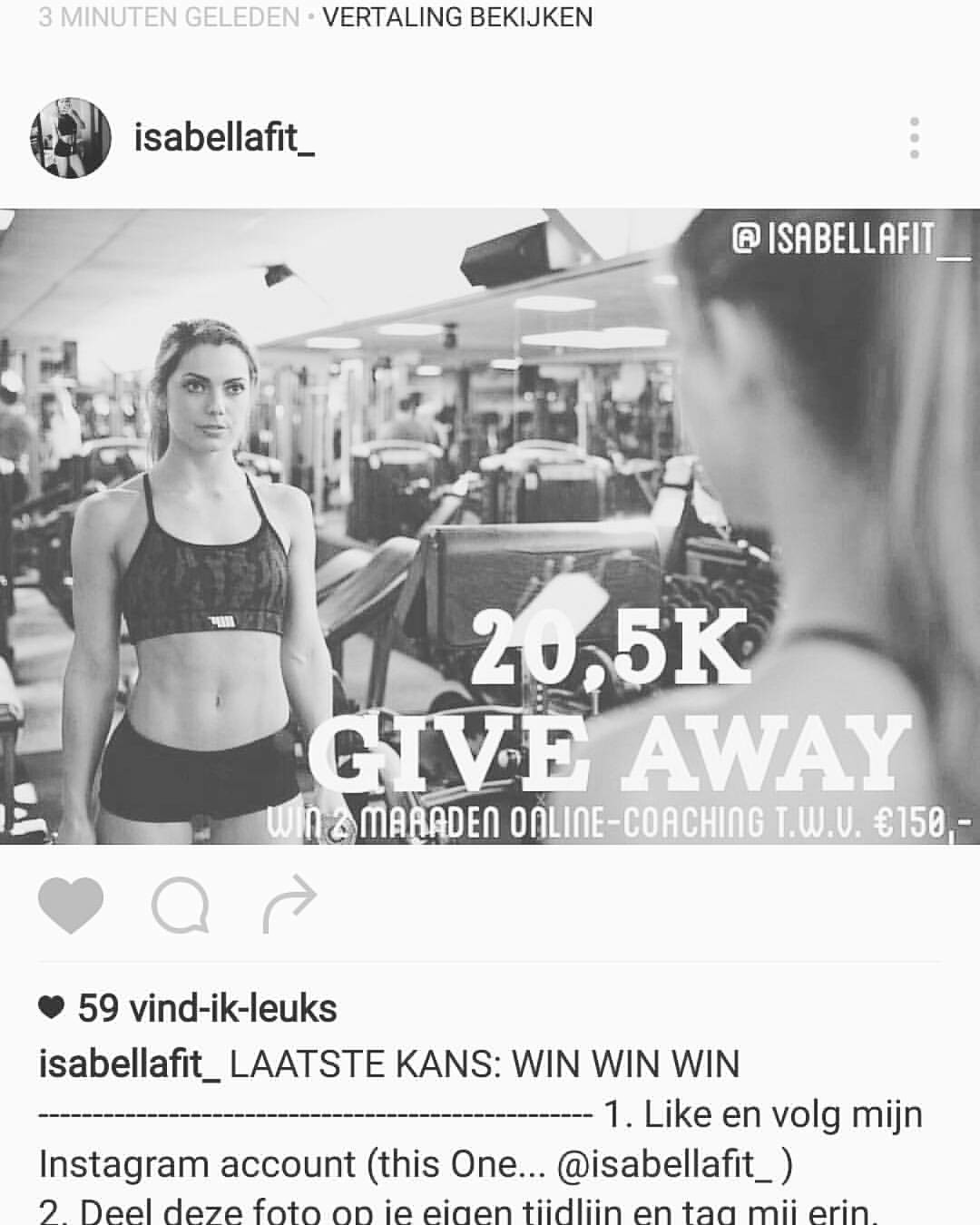Instagram post by IsabellaFit_ showcasing a black-and-white photo of a fit woman in a gym. The woman, dressed in a sports bra and shorts, is facing a mirror with her hair in a ponytail. Behind her, there's gym equipment, including a sit-up area, speakers, and some weights. The gym appears relatively empty, with maybe a few people in the background. Overlaying the photo is text that announces a "20.5k giveaway - Win online coaching valued at 150 euros." Below the image are Instagram interface elements, including heart, comment, and share buttons. The text beneath the buttons reads: "59 wind-ik-lux IsabellaFit_ last day chance win win win one like and Vogue Magazine Instagram account @IsabellaFit_." The entire screenshot is in black and white.